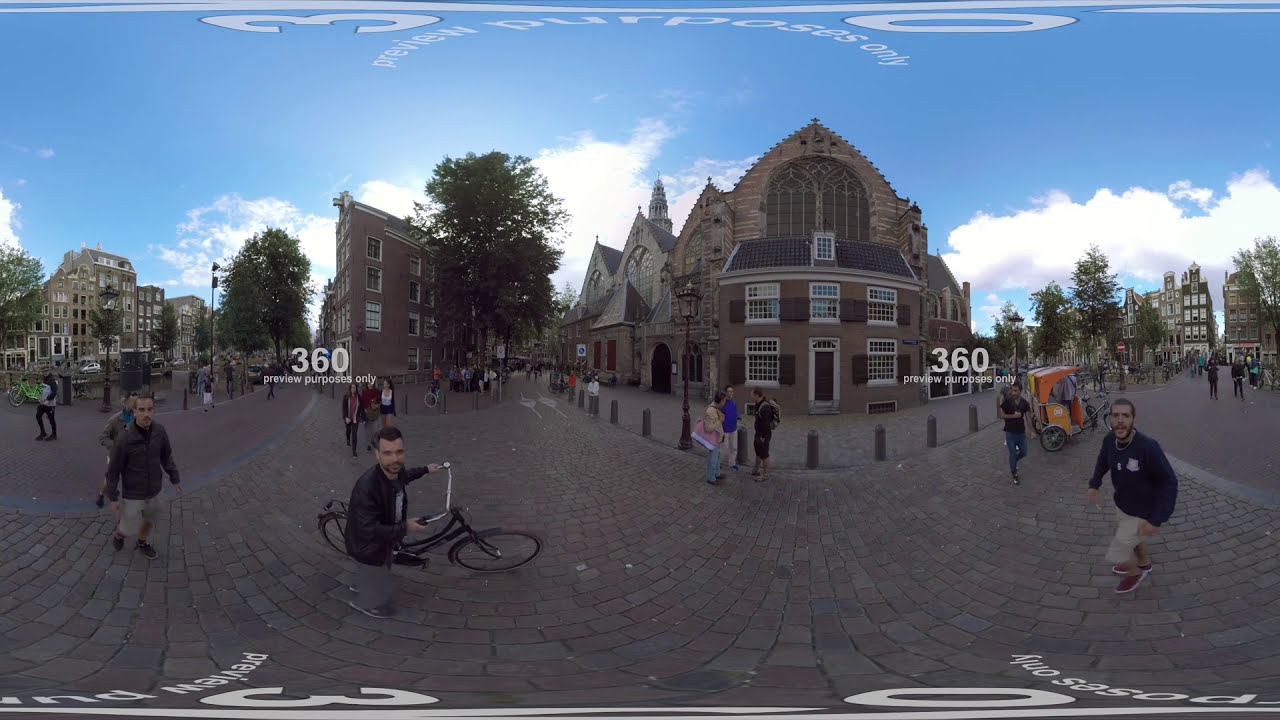An outdoor 360-degree panorama showcases a bustling scene in front of a grand, multi-story building with classical European architecture featuring ornate gables. The structure, constructed predominantly from old stone with red brick fronting, sits centrally in the photograph, bordered by a wide, reddish-brown brick walkway. This building's façade is adorned with white-trimmed windows and doorways, and closely resembles a cathedral due to its artistic design. In the immediate foreground, three Middle Eastern men, all sporting beards, dark blue or black jackets, and gray or khaki cargo shorts, walk along the walkway. Additionally, a man with dark hair and a mustache stands on the left side of the image next to his bicycle, also wearing a dark jacket. The background reveals a mixture of people, possibly tourists, strolling along, indicating a lively atmosphere despite the cool weather suggested by their attire. The sky above is a bright turquoise blue, dotted with fluffy white clouds. On both sides of the image, there are other architectural structures, each distinct yet harmonious with the central building. The vibrant natural light illuminates the scene, enhancing the image's clarity, and green trees can be seen in the further distance, adding a touch of nature. Text reading "360 preview purposes only" appears prominently on either side of the photograph, confirming its panoramic nature.